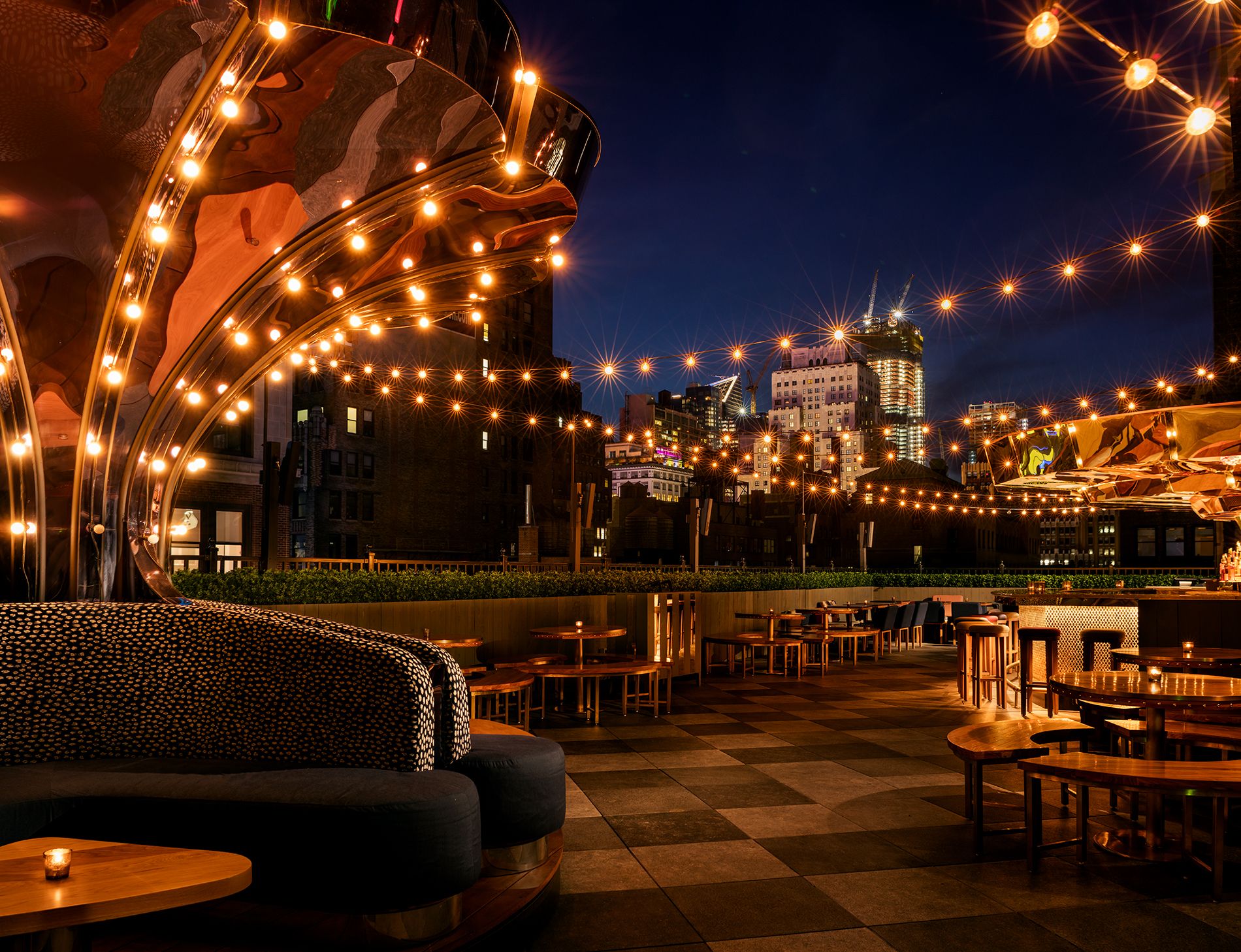This photograph captures a beautifully lit outdoor restaurant situated on a balcony against a picturesque nighttime cityscape. The setting exudes charm with its abundance of white draped string lights arcing across the space, casting a warm glow over numerous tables arranged on a black and white checkered tile floor. The tables are adorned with lit candles, enhancing the romantic and inviting ambiance. In the center, a bar area with modern stools beckons patrons who prefer a drink. Additionally, modern style couches and greenery add to the stylish and comfortable atmosphere. The backdrop features tall, illuminated skyscrapers, making this a perfect spot for a delightful dinner or a cozy evening with friends. The scene is devoid of people, making it a serene and immaculate visual of a perfect dining venue.